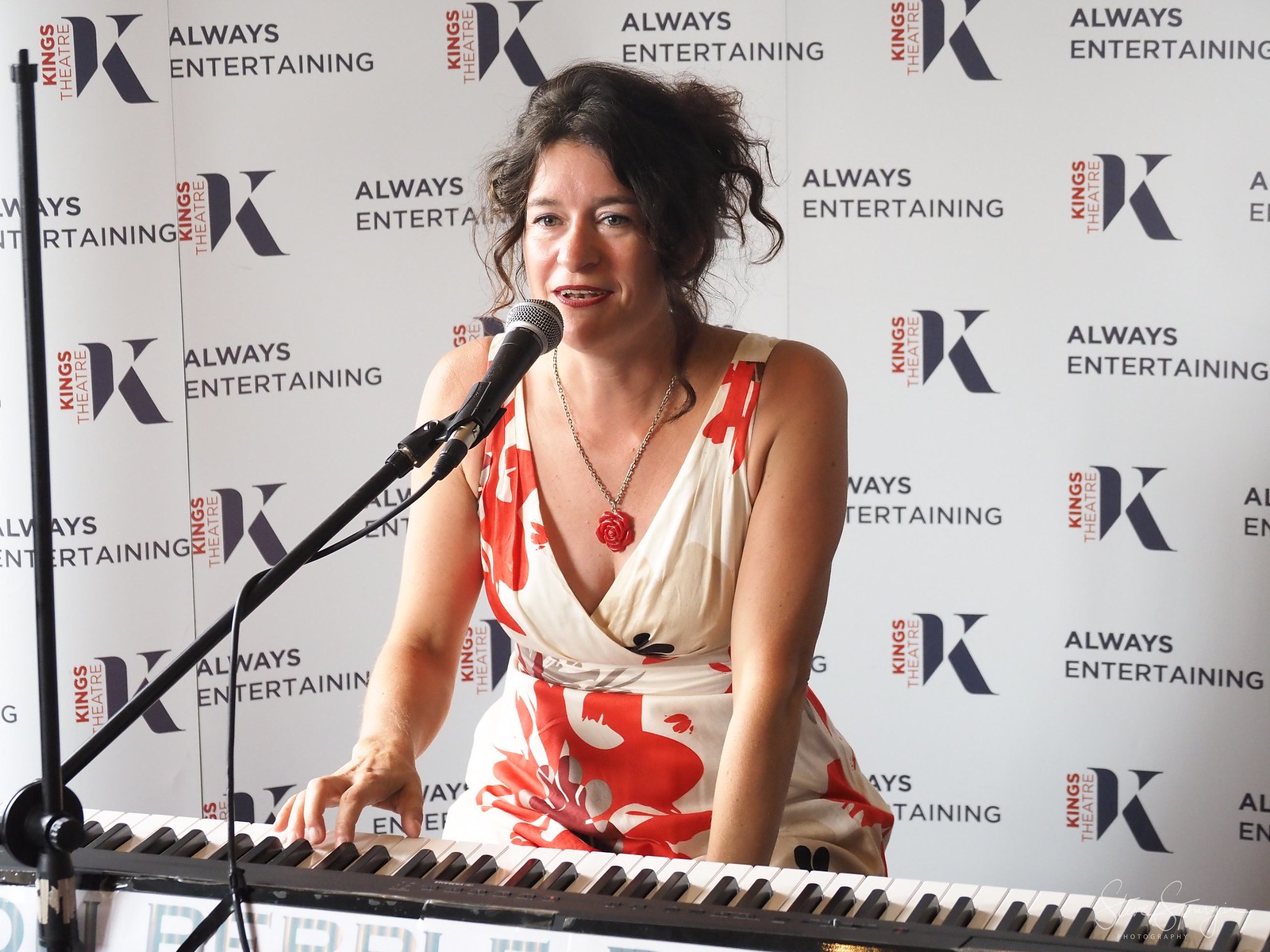In this detailed photograph, a woman in her fifties, with dark hair tied up in a bun, sits behind an electronic keyboard. She wears a cream-colored, low V-cut sundress decorated with scattered red patterns. Her right hand is on the keyboard, either pressing the keys or poised to do so, while her left hand rests beneath the keyboard. She appears to be mid-song, singing into a microphone that is positioned on a stand above the keyboard. Behind her is a large white wall adorned with a repeating pattern of logos and text that reads "King's Theater" and "Always Entertaining." The setup resembles a red-carpet photo spot, suggesting that this is an indoor performance at the King's Theater. The woman gazes slightly to the left of the camera, likely looking toward her audience.